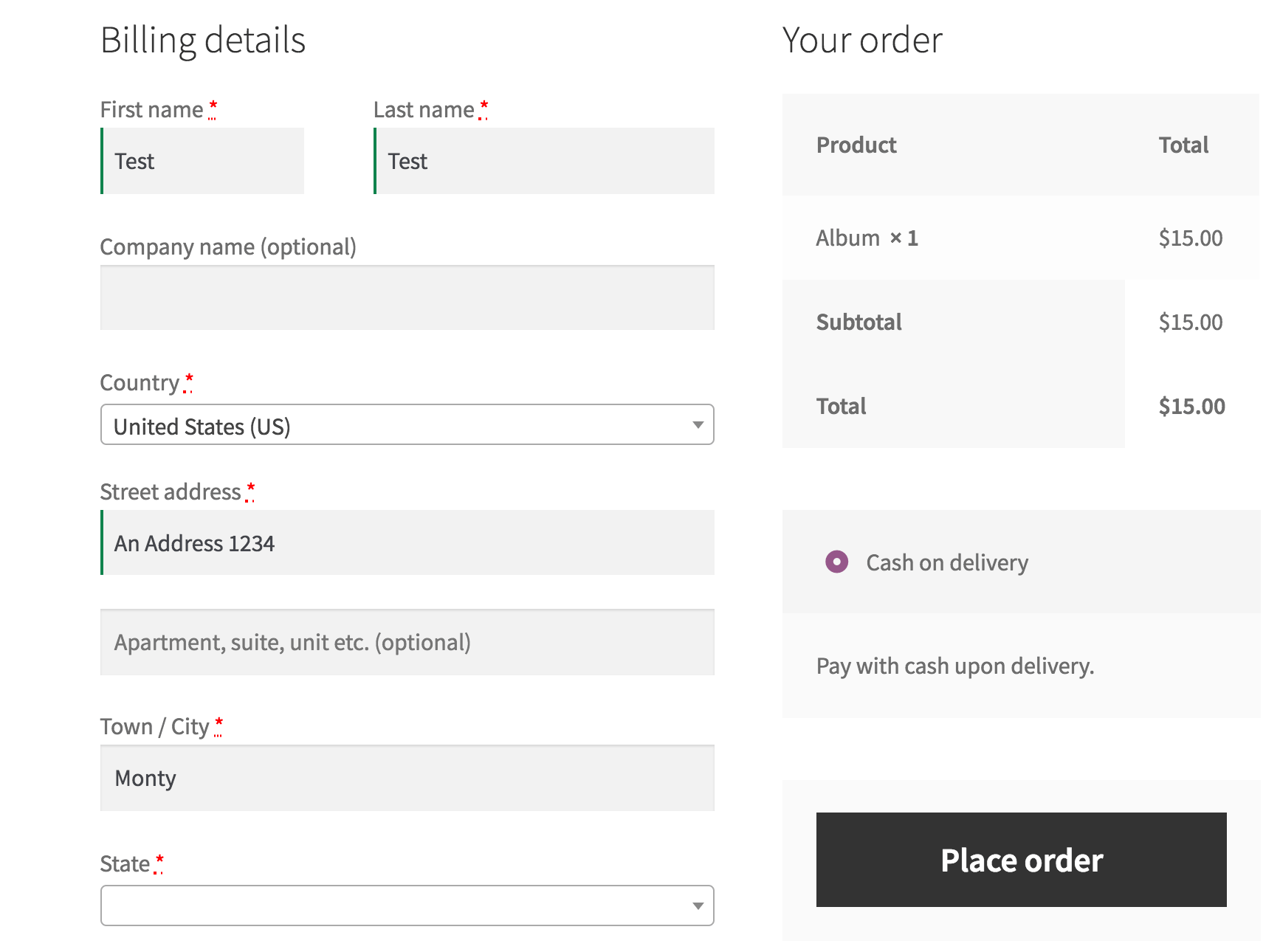Here is a cleaned-up and detailed caption for the described image:

"The screenshot features a form against a sleek white background, accented by gray and black text. At the upper left, 'Billing Details' is prominently displayed. The form includes fields for personal information: the first line has input boxes for 'First Name' and 'Last Name,' both filled with the placeholder 'Test.' Below that, there is an optional 'Company Name' field, followed by a dropdown menu for 'Country,' which is set to 'United States (U.S.).' Further down, there is a 'Street Address' field filled with '1234.'

On the right side of the image, an 'Your Order' section details the purchase information: a single 'Product' labeled 'Album' priced at $15. The 'Subtotal' and 'Total' both reflect this amount, listed as $15 each. Underneath, a light gray box indicates the payment method as 'Cash on Delivery,' with the note 'Pay with cash upon delivery.' Positioned at the bottom right is a large black 'Place Order' button, ready for action. To the lower left of this button is a form field for 'Town/City' and 'State,' completing the necessary details for the order.

Every element is designed with clarity and ease of navigation in mind, ensuring the form is user-friendly and straightforward."